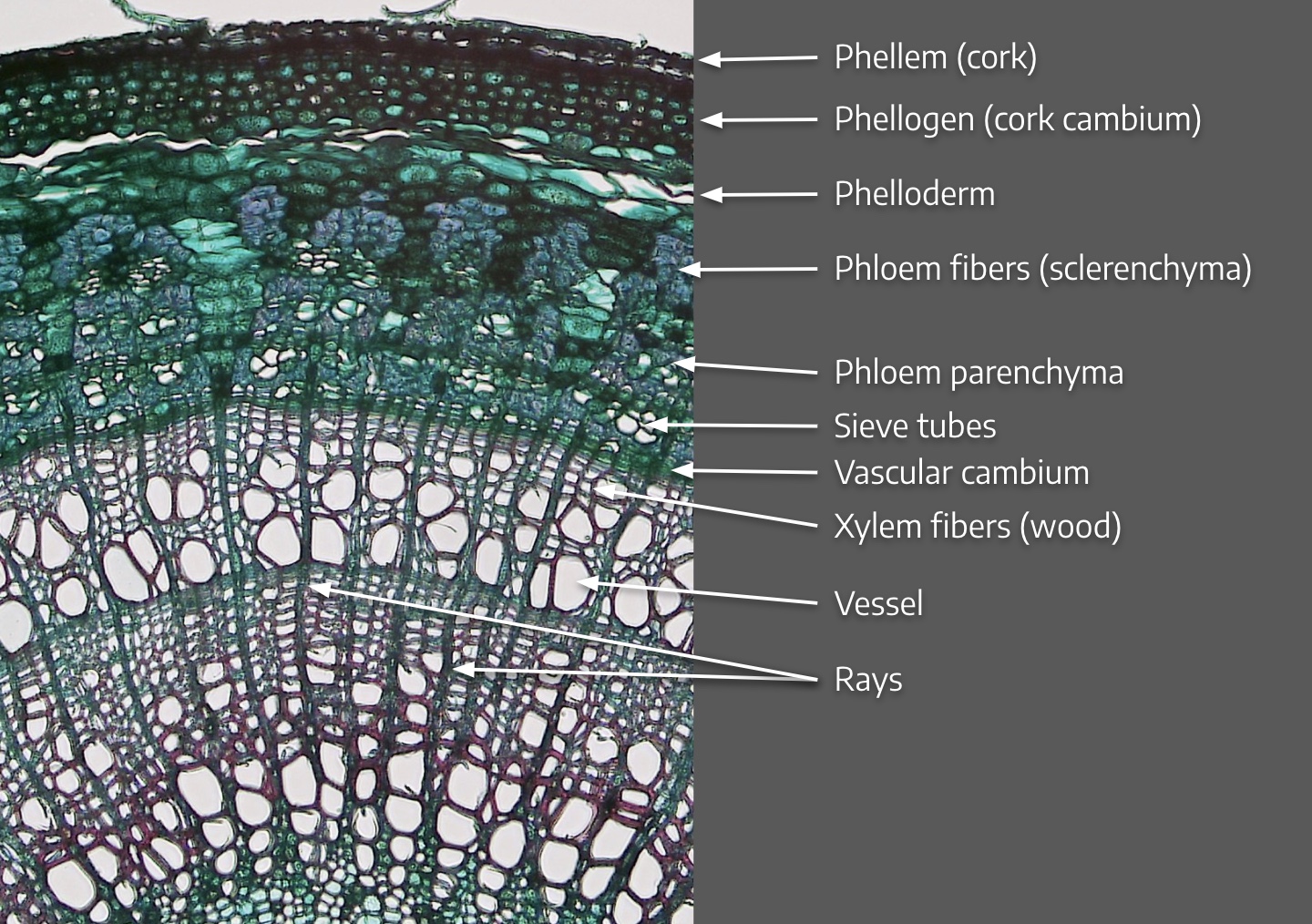The image presents a detailed scientific illustration, typical of those found in textbooks or scientific presentations. It is divided into two sections. The left side showcases a highly magnified view of cellular structures, resembling a doily with intricate patterns of fibers in vibrant greens, blues, and purples. These fibers and cell walls contribute to the overall complex texture of the microscopic organism. The right side of the image features a gray background with white text detailing various components, each labeled with arrows. The labels, arranged from top to bottom, include: "phyllum (cork)," "phyllogen (cork cambium)," "phylloderm," "phloem fibers (sclerenchyma)," "phloem parenchyma," "sieve tubes," "vascular cambium," "xylem fibers (wood)," "vessel," and "rays." This side clearly annotates the different parts of the cellular structure depicted on the left, making it a comprehensive visual tool for understanding the intricacies of the organism.